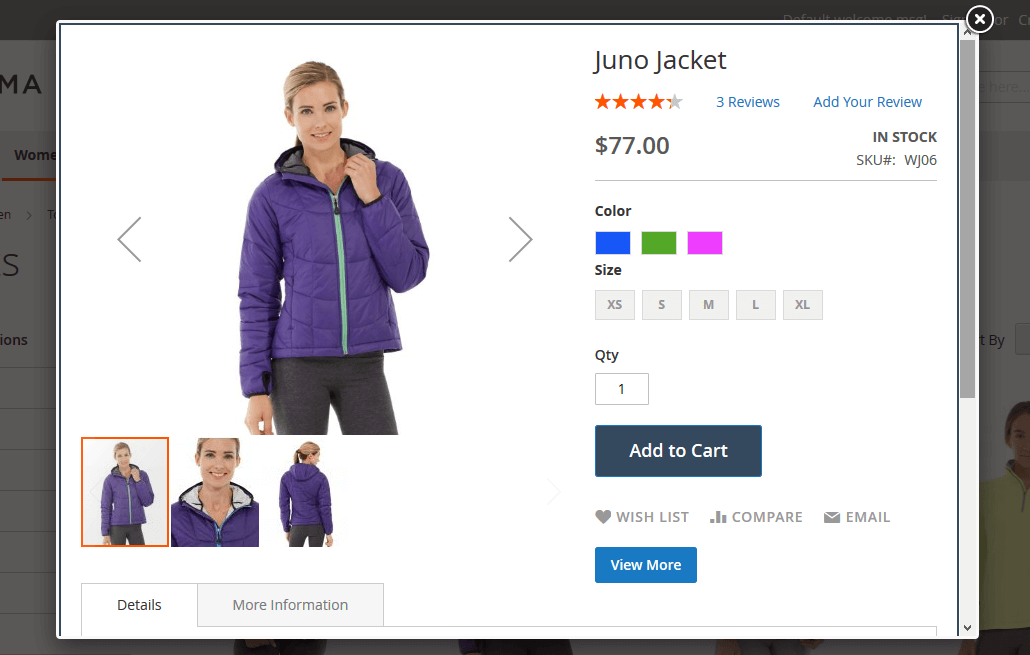Here is a cleaned-up and detailed caption for the image described:

---

This image is a detailed screenshot from an online shopping website, focusing on a pop-up product window that has taken center stage. The background is slightly blurred with a dark shadow effect, allowing the pop-up to stand out clearly. At the top-right corner of the pop-up, there is a small circle with an 'X' for closing the window.

The product displayed is the "Juno Jacket," which has a rating of about four out of five stars based on three reviews. There is an invitation to "Add Your Review" beside the rating section. Below the rating, the price of the jacket is listed as $77. On the right side, it is indicated that the item is "In Stock" with an SKU number of WJ06. 

Color options are displayed beneath the SKU number, featuring three rectangular swatches: blue on the left, followed by green, and then magenta. Size options are provided in five grayed-out rectangles labeled XS, S, M, L, and XL, suggesting that either no size has been selected yet or sizes might be out of stock. Below the size options, there is a quantity (QTY) text box set with the number 1. 

The "Add to Cart" button is prominently placed beneath these options. Further down, there are additional buttons for "Wishlist," "Compare," and "Email," followed by a "View More" button.

On the left side of the pop-up, a model is featured showcasing the jacket. She has her hair tied back and is wearing the purple puffy "Juno Jacket" paired with gray leggings. Below her photo, there are three small thumbnails of different images of the model displaying the jacket from various angles.